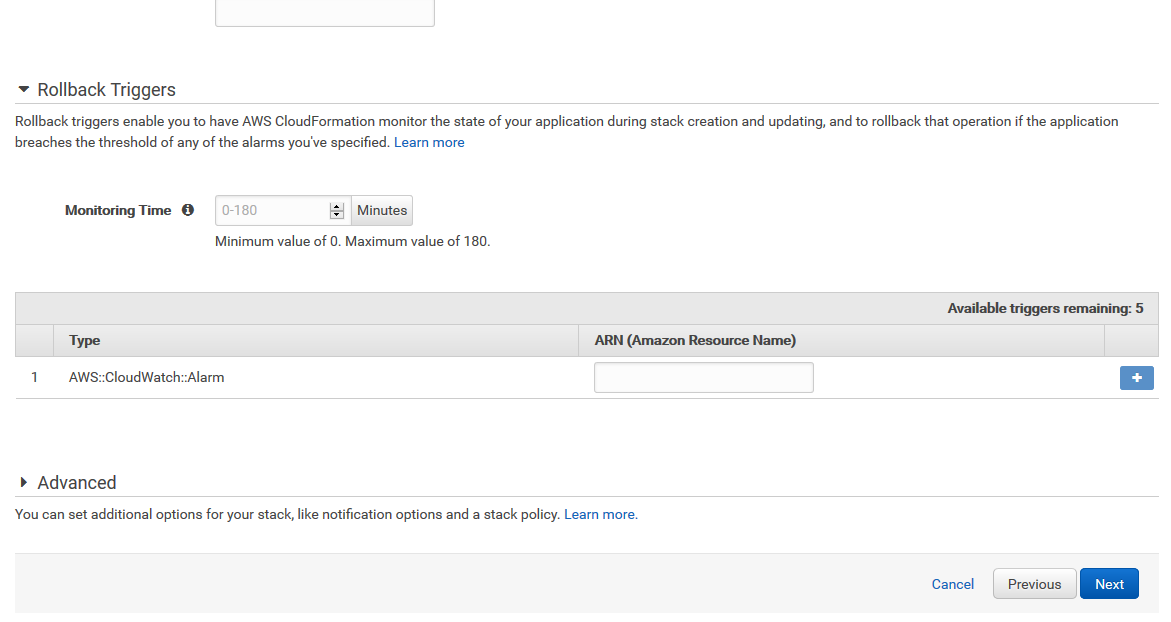The image showcases a detailed interface from AWS CloudFormation, primarily focusing on rollback triggers for monitoring application state during stack creation and updates. 

At the top, there is a drop-down box labeled "Rollback Triggers." It explains that rollback triggers enable AWS CloudFormation to monitor the state of an application during stack creation and updating, rolling back the operation if the application breaches any specified threshold alarms. There is an option to learn more about the feature by clicking a button. 

Below, a monitoring time is displayed, which can be adjusted from 0 to 180 minutes via a user interface control. 

Further down, a gray bar indicates there are 5 available triggers remaining. The type is specified as "ARN" (Amazon Resource Name), with the first item being an "AWS CloudWatch Alarm." The interface also allows users to add more triggers by clicking.

Additionally, there is a section labeled "Advanced," where users can configure further options for their stack, including notification settings and stack policies, with more information accessible through a clickable link.

The lower part of the interface presents navigation options labeled "Cancel," "Previous," and "Next," aiding users in navigating through the setup process. The overall context suggests that users are in the midst of configuring their application stack on AWS CloudFormation.